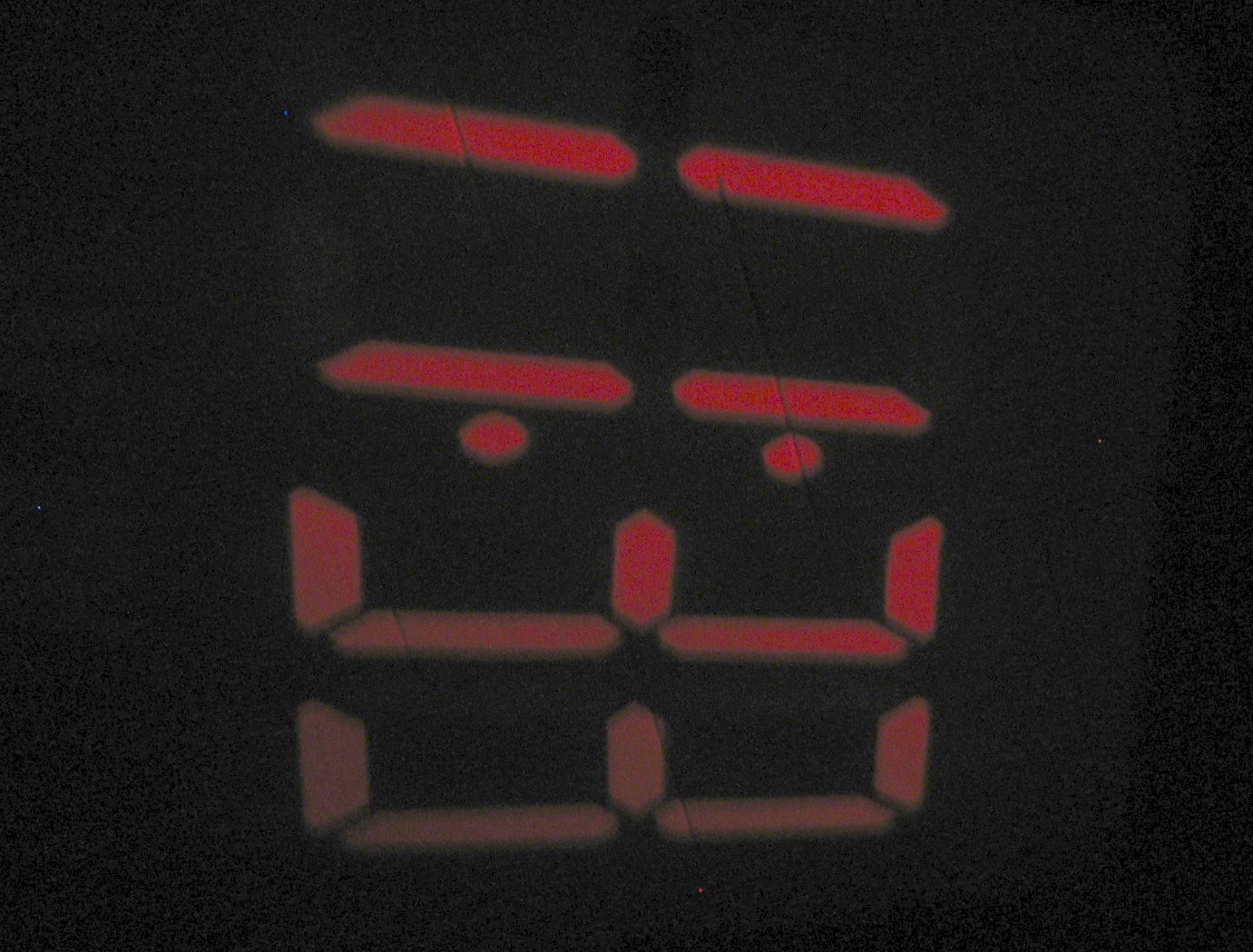In this rectangular image, there is a close-up view of a digital clock display set against a solid black background. The numbers are oriented sideways, with the top of the clock on the right and the bottom on the left. The digital display reads "1133". The "11" is prominently lit in a bold, vibrant red color, making it stand out significantly against the black backdrop. In contrast, the "33" appears much dimmer and less defined, with a far-shaded and duller red hue. The two dots separating the "11" and the "33" are illuminated in the same bright red as the "11", adding a striking focal point to the image.